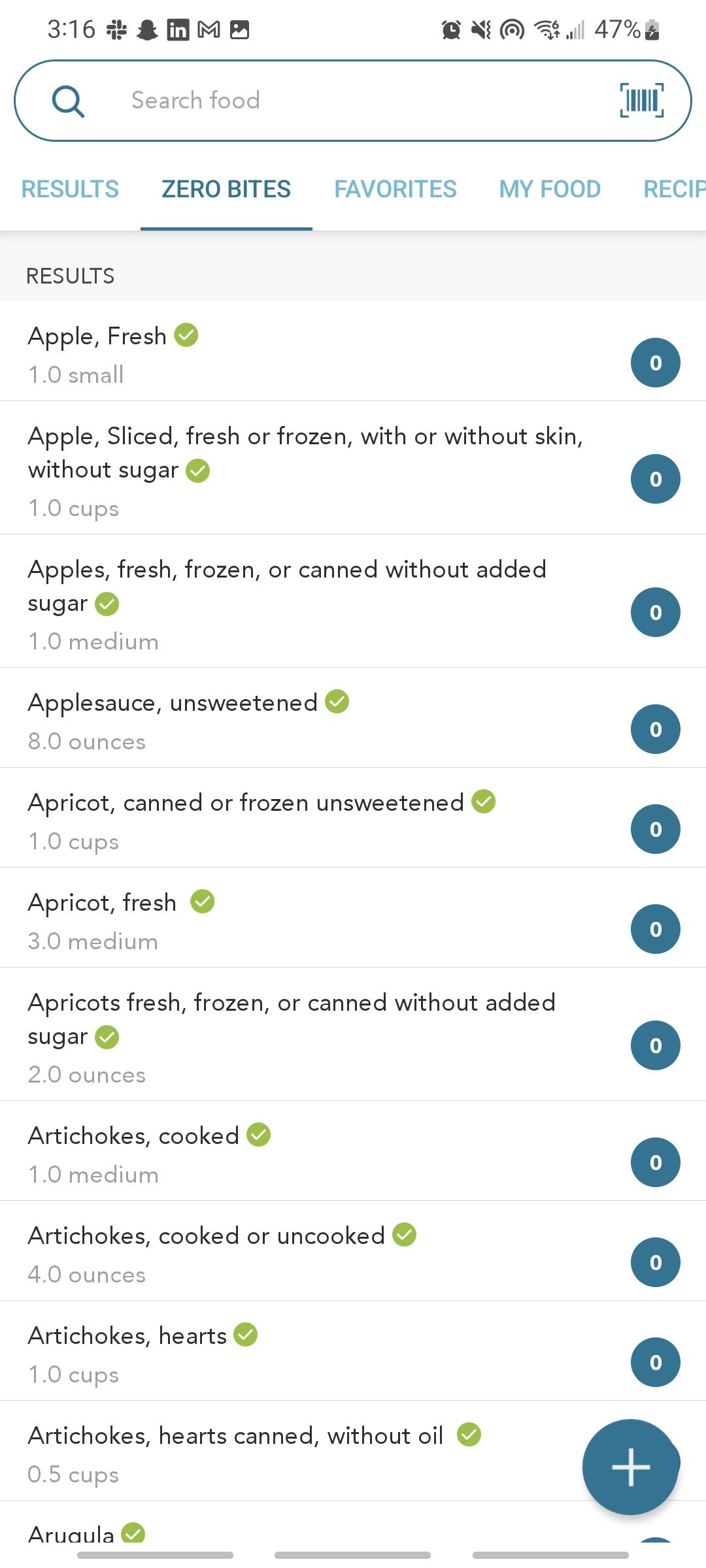The image displays a smartphone screen showcasing a website interface. At the top of the screen, the status bar reveals essential phone details: a battery at 47%, sound is muted, good network connectivity, and the time is 3:16 PM. 

Directly below the status bar is a search bar where the term "food" has been entered. Beneath the search bar, navigation options such as "Zero Bites" (highlighted in blue with a bar underneath), "Favorites", "My Food", and "Recipe" (partially cut off and likely meant to read "Recipes") are visible.

The search results are displayed in a gray bar below the navigation options. The list of food items includes:
- Apple, fresh
- Apple slice, fresh or frozen, with or without skin, without sugar
- Apples, fresh, frozen, or canned, without added sugar
- Applesauce, unsweetened
- Apricot, canned or frozen, unsweetened
- Apricot, fresh
- Apricots, fresh, frozen, or canned without added sugar
- Artichokes, cooked
- Artichokes, cooked or uncooked
- Artichoke hearts, canned without oil
- Arugula

The screen cuts off at the end of the "A" section of food items, suggesting that more results could be visible by scrolling further down.